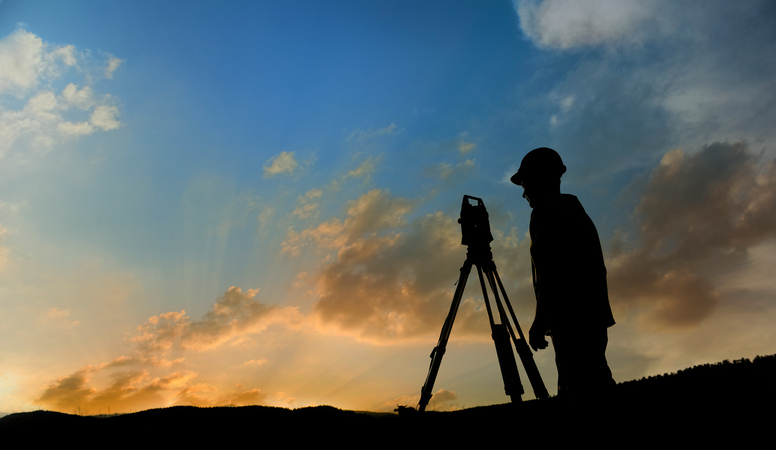The photograph captures a striking silhouette of a man, likely a land surveyor, standing on a high, sloped surface at sunset. The man, wearing a jacket, pants, and a construction hat, is positioned on the right side of the image with a camera or surveying instrument mounted on a tripod before him. The scene is cloaked in shadow due to the low sun, creating an almost ethereal quality. The sky unfolds above in a gradient of deep blue at the top, transitioning through white clouds to darkening hues closer to the horizon, where the clouds are tinged with yellow and pink. The land beneath him appears dark, contrasting sharply with the vibrant, colorful sky illuminated by the setting sun's rays. Though the details of the instrument remain indistinct due to the silhouetted light, the overall composition exudes a sense of solitude and purpose, capturing the stark beauty of the sunset against the twilight landscape.